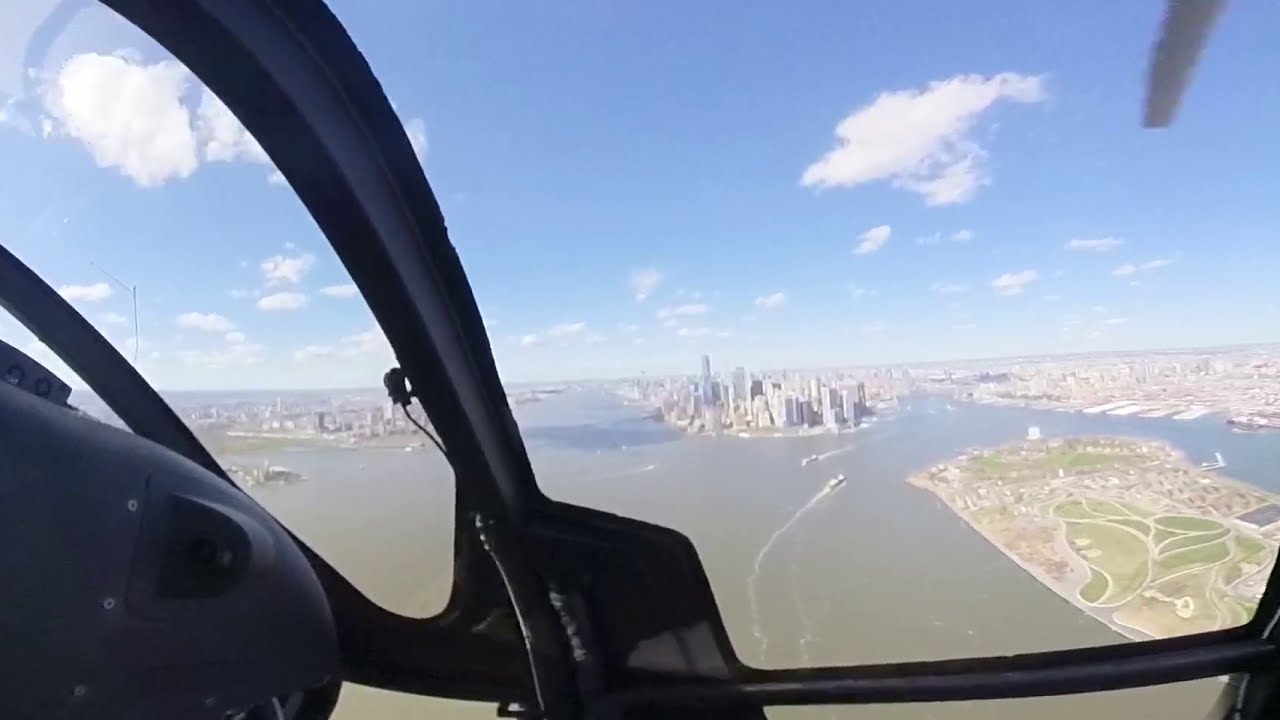This highly detailed aerial photograph captures an expansive view of a city, likely Manhattan, as seen from the cockpit of a dark green helicopter, with its distinct windshield framing the shot. The helicopter hovers over a vast expanse of blue water, where a few boats leave visible trails behind them. In the distance, the densely crowded cityscape rises with numerous tall buildings, suggesting it's a major urban area situated on an island. To the right of the frame, there is a prominent green park area, surrounded by streets and smaller structures. The sky above is clear blue adorned with white clouds, enhancing the vivid daytime scene.